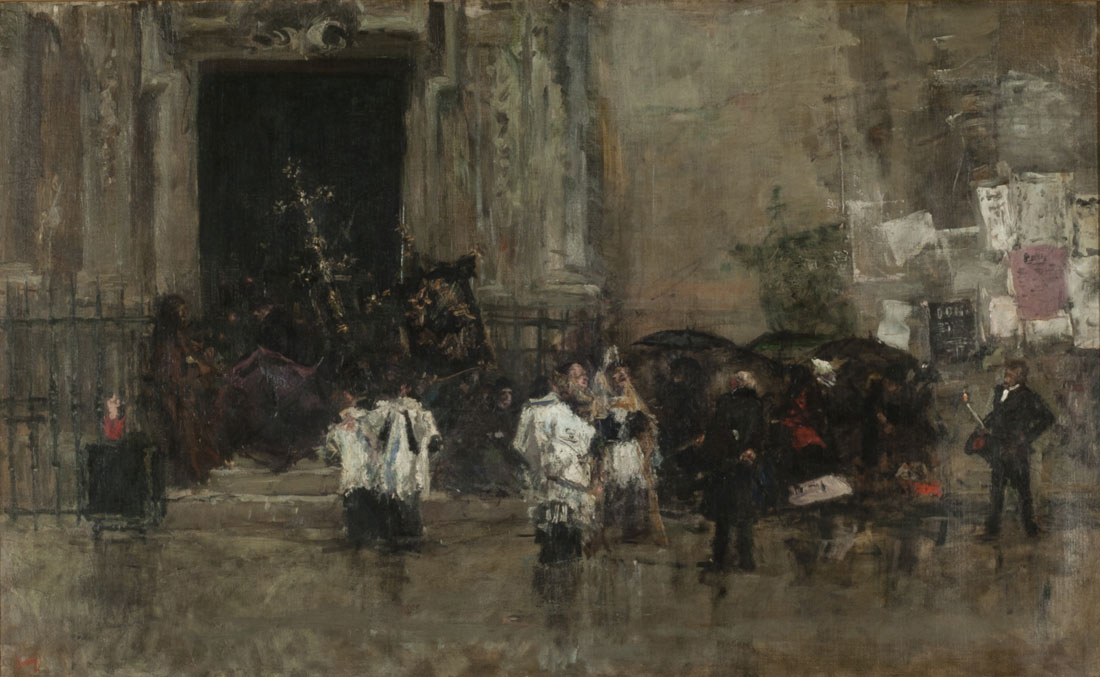This image is a painting that gives an impressionistic, somewhat blurry view of a city street scene, possibly painted in watercolors. Dominated by thick, smeared brushstrokes, the painting exudes a gray and muted tone, with hints of white, black, red, and gold peeking through. The main focus is a tall, stone-like building with a massive doorway toward the left. The door is almost engulfed in darkness, accompanied by a metal fence on both sides. 

In front of this grand entrance, which resembles that of a cathedral or a church, stands a gathering of people. To the left of the scene, people dressed in white shirts and black pants are visible, possibly altar boys or priests. Closer to the right bottom part of the image, there is a distinct figure of a man in a black suit with a white undershirt, engaged in what seems like moving a large, ornate chandelier or painting through the doorway.

Above this man, various notices and pieces of paper in white, pink, and black cling to the building's side, creating a board of sorts. The street below is depicted with a mirror-like, cobblestone effect in hues of brown and tan, suggesting a textured, reflective surface. This street activity, likely set during the fall or winter months and possibly taking place during the day, captures the bustling movement and preparations of the individuals. The overall scene, with men in black suits possibly holding canes or instruments, carries a solemn, yet vibrant energy, reflective of an urban place with historical resonance.